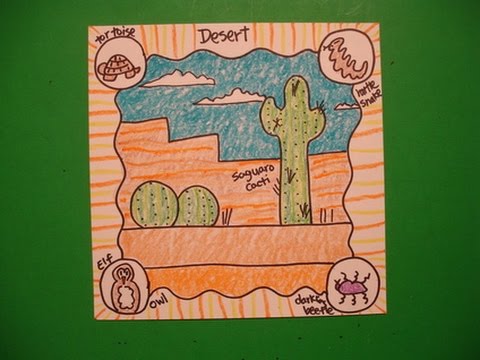This image features a hand-drawn depiction of a desert landscape on a green background, likely created by a teenager or child. The drawing, framed by alternating orange and yellow lines, prominently displays the word "desert" at the top. In each corner, there are labels and illustrations of desert animals: a tortoise in the upper left, a snake in the upper right, an elf owl in the lower left, and a darkling beetle in the lower right. The center of the drawing showcases a blue sky with white clouds above a stepped desert terrain, which includes a large saguaro cactus labeled "Saguaro Cactus" and two smaller round cacti. The scene is detailed with brown earth tones below the cacti, creating a vivid desert environment.